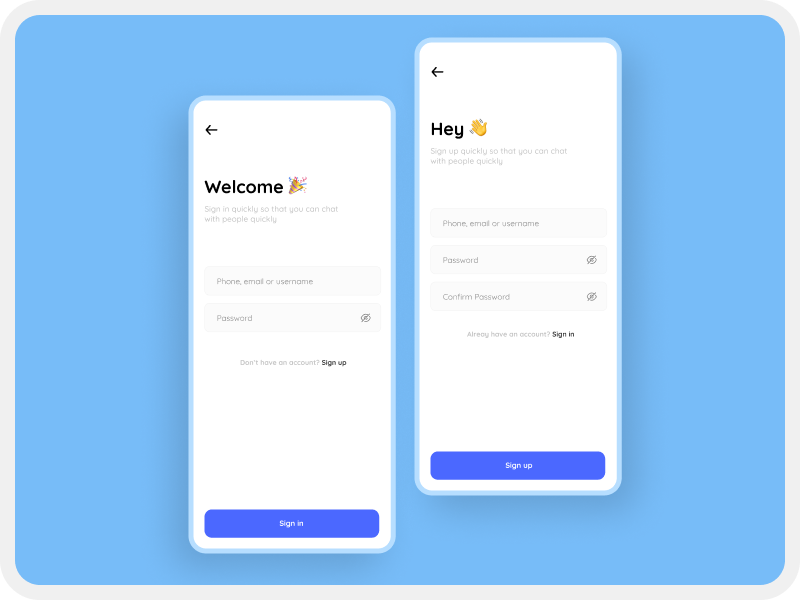This image features a large, blue rectangle with rounded edges and a white border. Within the blue area are two illustrations of smartphones displayed face-up, each with a white screen. The smartphone on the left welcomes users with a message that includes the party confetti emoji and prompts them to sign in to chat with people quickly. The sign-in interface includes fields for phone, email, or username, and password, as well as a prompt for those who do not have an account to sign up. A 'Sign In' button is located at the bottom of the screen.

The smartphone on the right greets users with a 'Hey' message accompanied by the waving hand emoji and encourages them to sign up to chat with people quickly. The sign-up interface includes fields for phone, email, or username, password, and confirm password, along with a prompt for those who already have an account to sign in. At the bottom of this screen is a 'Sign Up' button housed inside a dark blue rectangle. The entire image lacks any photographic elements, people, animals, birds, plants, flowers, trees, buildings, mountains, automobiles, motorcycles, and bicycles, making it a purely illustrative and text-based depiction.